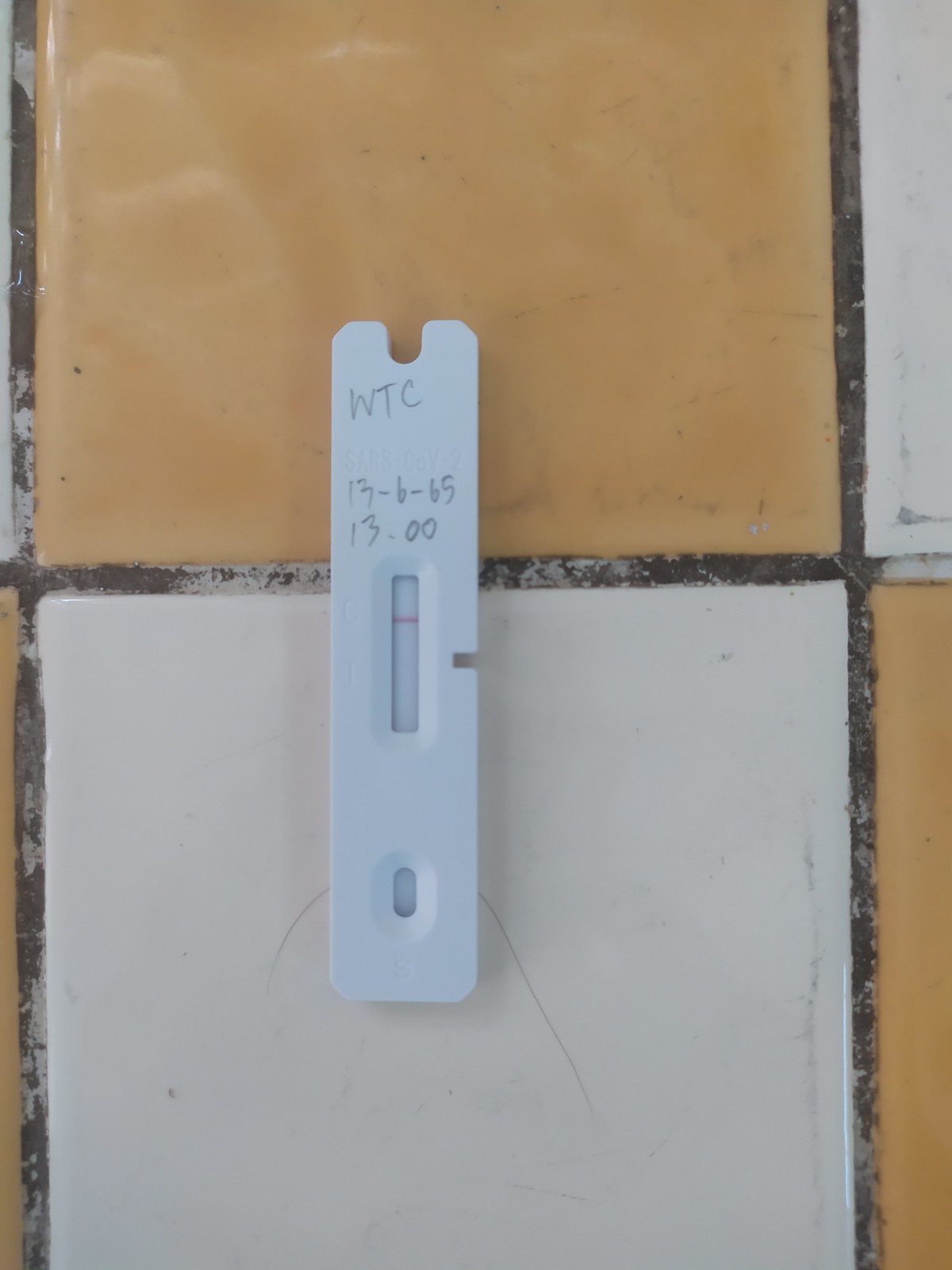This photograph features a white plastic at-home test, which could be either a pregnancy test or a COVID-19 test. The test is placed upright on a surface of alternating white and orange square tiles, with visibly discolored gray grout, indicating the tiles are quite aged. The test itself bears several inscriptions: "WTC," "13-6-65," and "13.00." A small window near the top of the test shows a single line positioned about a quarter from the top edge, while below it is an opening meant for applying the sample, whether it's urine or nasal swab. Additionally, a black hair is noticeable on the tiles, situated between the tiles and the test, adding an element of randomness to the scene.